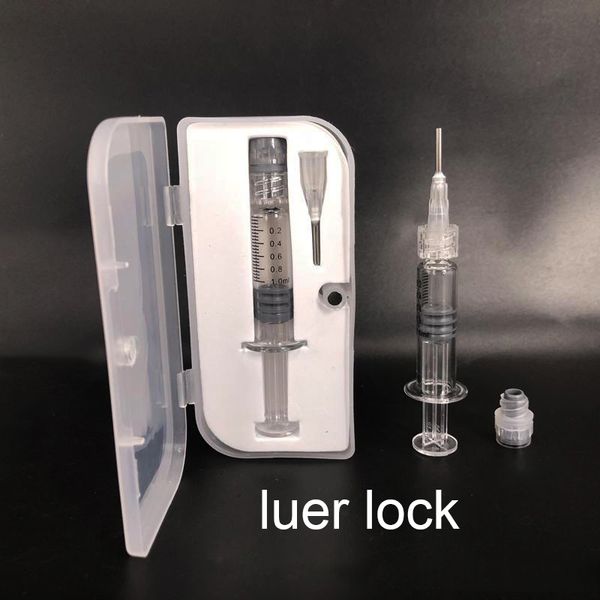The image depicts a detailed view of a medical setup featuring a hypodermic syringe kit contained in a clear plastic case positioned upright and open. The case, lined with white padding, securely holds the separate components of the syringe, including the syringe body with fill level markings and the corresponding needle tip housed in tailored slots. To the right of this case lies a fully assembled, transparent hypodermic syringe with its needle attached and a small cap placed further right. Both syringes exhibit fine metal needle tips. The background of the image is gray and blurred, creating a stark contrast with the items, which rest on a dark surface. Beneath the case and syringe, the term “Luer lock” is prominently displayed in white, lowercase letters, indicating the type of connection system for the syringes.